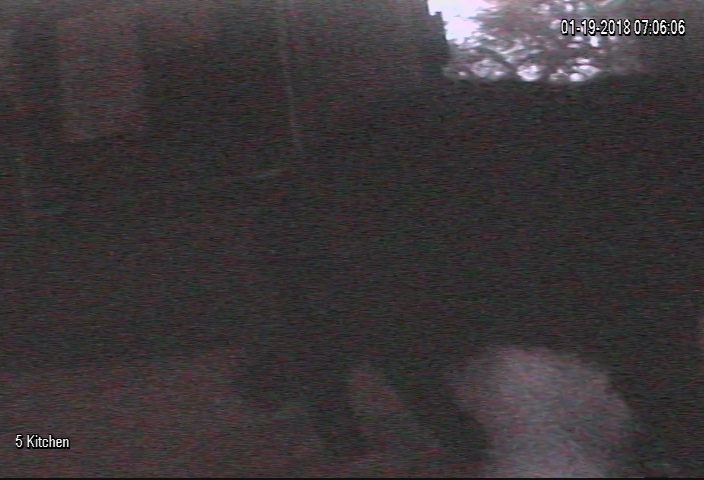In this nighttime photograph taken on January 19, 2018, the scene is dimly lit and slightly blurry. The focal point appears to be a small dog standing on a sidewalk. The animal is discernible by its four short legs. The ground is paved with reddish, brick-shaped stones interspersed with a few darker ones, creating a muted pattern in the scant light. In the background, a building is partially visible, with windows that reveal nothing from their darkened interiors. To the right of the building, a fence extends into the distance, beyond which trees are faintly outlined by a soft illumination. The left side of the image is enveloped in darkness, with only a few elements on the right side faintly discernible due to limited lighting. The timestamp "5 Kitchen" is displayed at the bottom, indicating a recorded time associated with this enigmatic outdoor scene.